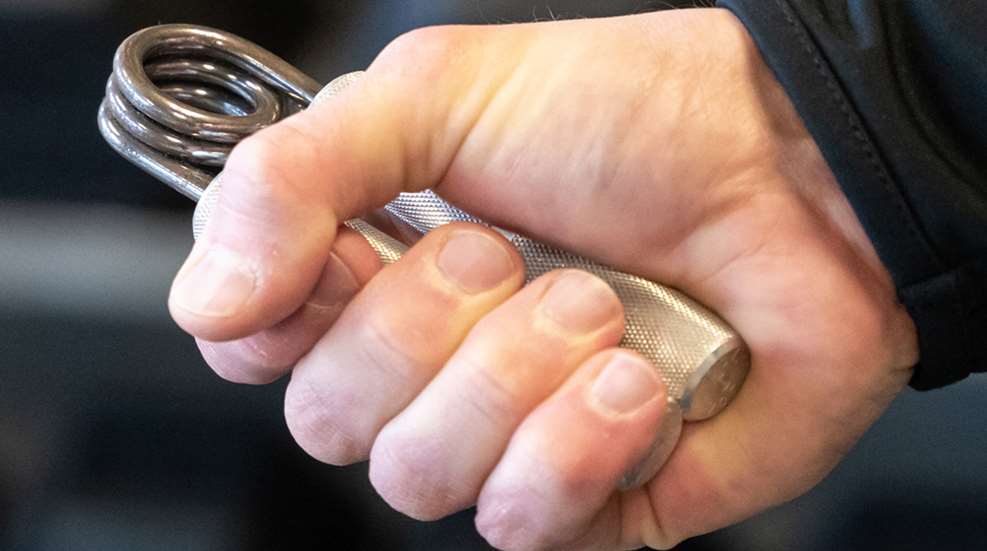In this image, a Caucasian person is using a hand grip strength tool. Their hand, which is bulky and thick-fingered, firmly squeezes the tool's brushed silver metal handles. These handles feature a grippy texture comprising lines and dots. The device's top showcases a shiny chrome coil arranged in a spiral design. The user is attired in a black, long-sleeved jacket, possibly made of polyester. The background is mostly gray and blurry, making it hard to discern specific details beyond the hand and the exercise tool.